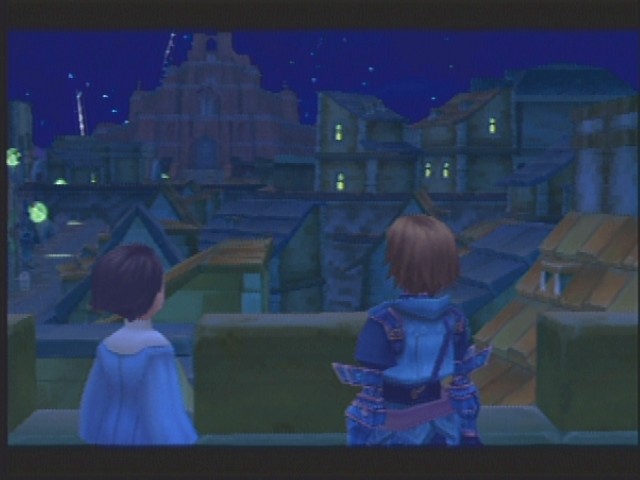In a captivating animated scene, two characters stand on a balcony, their backs to the viewer, gazing out at an intricately detailed medieval-style town under a starry night sky. One character, with bright brown hair, donned in medieval armor, stands to the left. Beside them, a figure with dark brown or black hair, wearing a blue long-sleeve garment with a distinctive white collar that hints at period attire, completes the duo. The town below is vibrant, with buildings illuminated by yellow lights peeking through windows, casting a warm glow against the blue, green, and orange hues of the scene. Dominating the center, an imposing brown castle rises among triangular-roofed structures, adding to the town's historic charm. The entire image is framed by black strips on the top and bottom, adding a cinematic feel, though it could be from a game or a digitally drawn artwork.